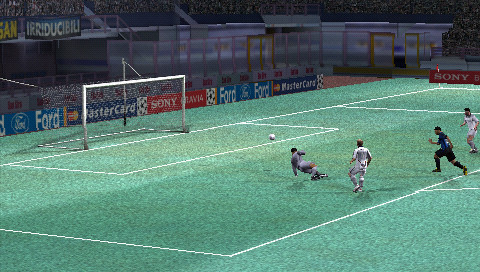This rectangular image, oriented horizontally from left to right, captures a dynamic moment on a soccer field. The scene's nature is ambiguous, blurring the lines between reality and a computer-generated snapshot. At the heart of the action are four players in full sprint, with the soccer ball seemingly propelled towards the goal. The precise origin of the kick and the location of the goalie remain unclear. The vibrant green field features distinct white lines marking the goalie box and the penalty area. Prominently, the goal itself has a white crossbar and upright posts, framing a tense focal point of the game. A corner flag is situated in the upper right corner, adding a touch of authenticity to the setting. Surrounding the pitch, a series of advertisements line the edges, each promoting various brands and products, lending a sense of immersion to the scene.